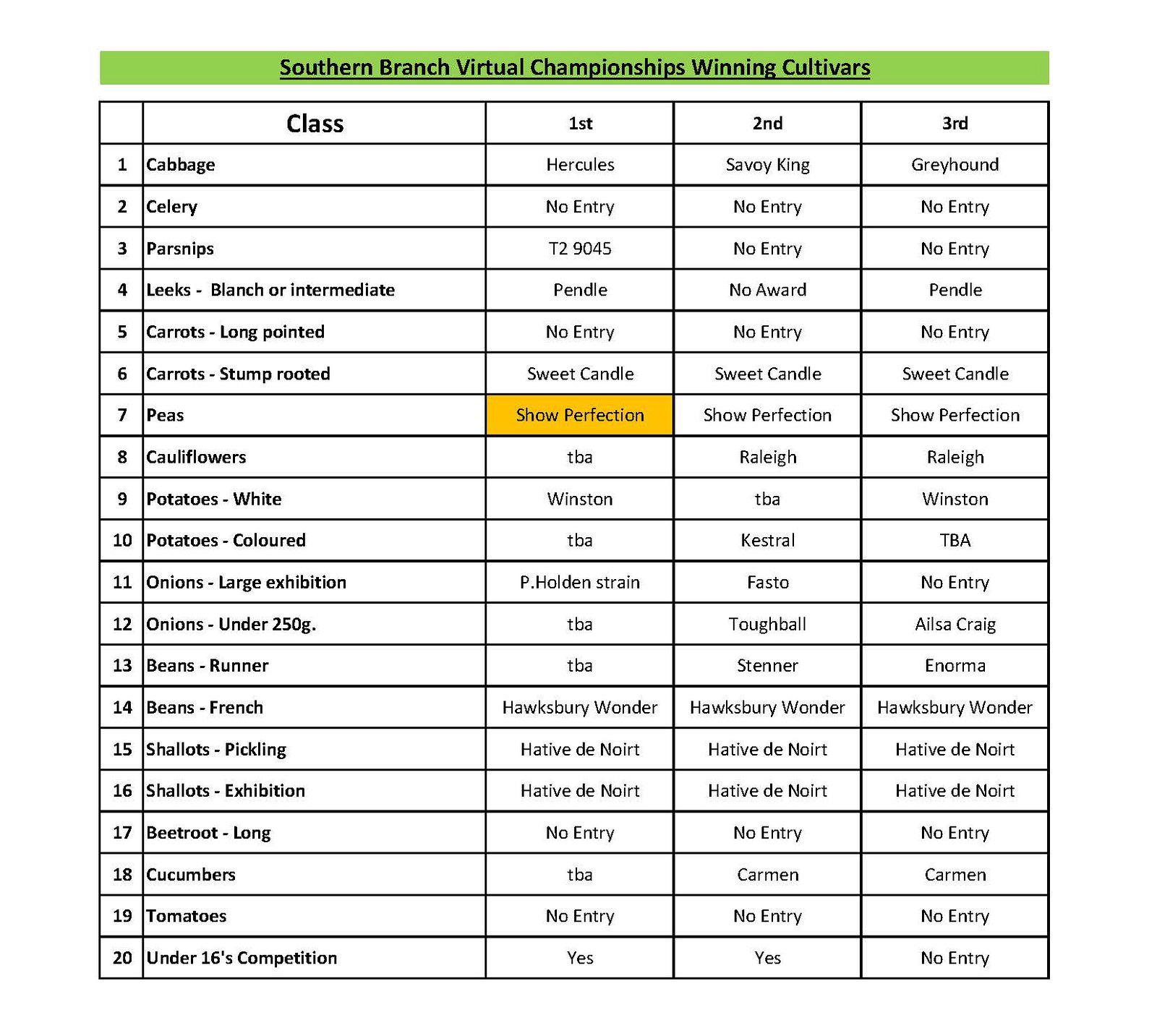The image depicts a detailed table diagram in a black and white print publication with spot color accents, specifically in lime green, orange, white, and black for the text. This square format print, likely created for an advertisement or informational chart, is titled "Southern Branch Virtual Championships Winning Cultivars" prominently displayed in a light green horizontal strip across the top. The table features 20 rows numbered 1 through 20 in the leftmost column. The second column, labeled “Class,” lists various crop categories such as cabbage, celery, parsnips, leeks, carrots (both long pointed and stump-rooted), peas, cauliflowers, white potatoes, colored potatoes, onions, beans, shallots, beetroot, cucumbers, tomatoes, and a special under 16 competition. The subsequent columns are headings for 'First', 'Second', and 'Third' places, with varying entries under each crop category. Notably, the seventh row features a gold-highlighted box with the text "Show Perfection." The overall style is reminiscent of organized print collateral, designed for easy readability and visual appeal.